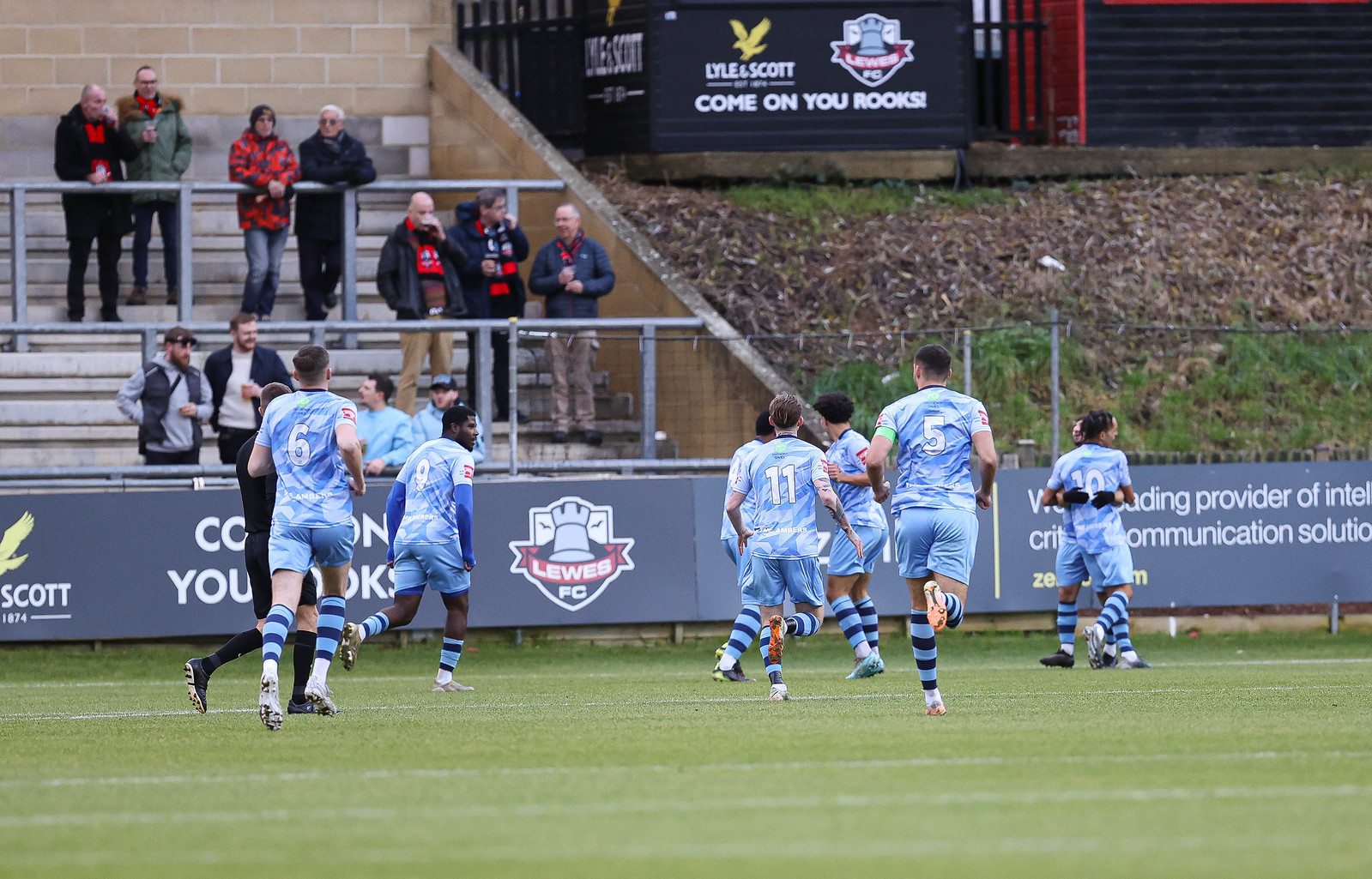In this detailed outdoor image of a soccer match, the team in focus is dressed in light blue jerseys and shorts, with blue and dark blue striped socks. Visible numbers on their backs include 5, 6, 11, 10, and potentially 8 or 9. The players are actively moving across a level green field, with some hugging each other, capturing a moment of camaraderie. 

In the foreground, the lush green of the field stands out, while the midground features a border area adorned with advertisements and a blue backdrop. To the left of this border, bleachers are visible with a few spectators standing and leaning against the bars, intently watching the game. The atmosphere suggests a relaxed crowd, not densely packed.

Further to the left beyond the bleachers, the terrain inclines upward, revealing patches of grass and dirt. In the background, several signs are visible. Prominently, "Come on, you rooks" and "Lyle and Scott" are written on signage positioned towards the top right. Additional signage in the bottom right corner adds to the array of advertisements surrounding the field. A blank space in the top right area suggests a spot designated for yet another ad, mirroring the other areas' layout.